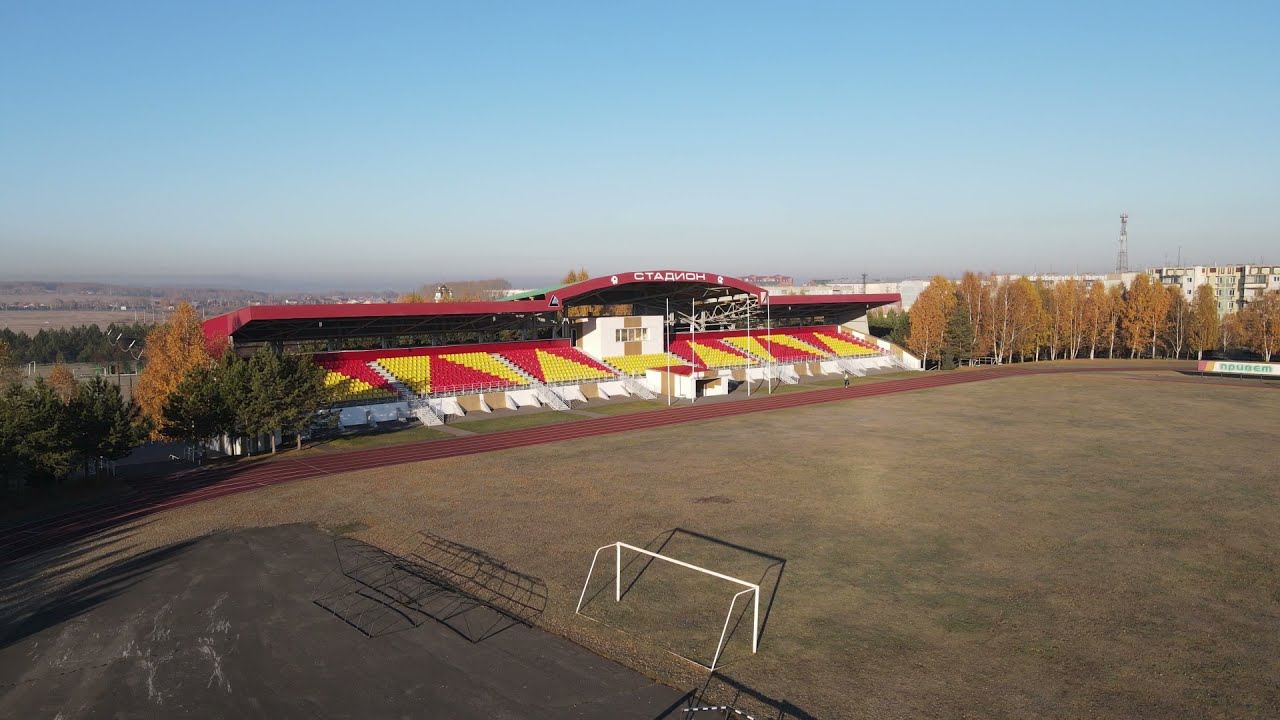The photograph captures a bright clear day in the autumn, featuring a large soccer stadium set in another country. The central focal point is a soccer field, where the grass has mostly turned brown, giving way to dirt patches. A striking red track encircles the field. Surrounding the stadium are stands with a colorful arrangement of red and yellow triangular patterns on the seats. Above the bleachers, an arch displays the text "GTAMANOH". White goalposts are situated at either end of the field, although the nets are absent. White walls frame part of the stadium area. In the distance, autumnal orange trees line the perimeter, and numerous 4-5 story buildings, possibly apartments or offices, along with a large power pole, add to the urban backdrop. The photograph, likely taken from a drone a few hundred feet above, beautifully captures the expansive layout and the vivid details of the stadium and its surroundings during the daytime.